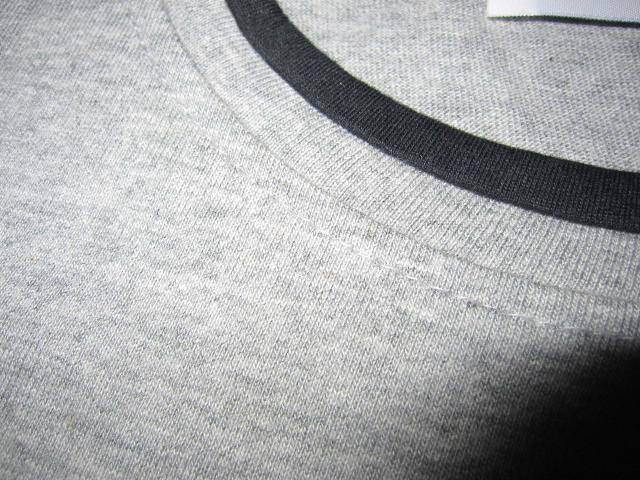This close-up image captures the intricate detailing of a heavy, knitted gray sweater, focusing specifically on its left upper collar area. The thick, textured knit of the sweater is prominently displayed, revealing varied tones of gray interspersed with slightly darker threads. The collar itself is substantial, consisting of two distinct sections: the main part, which shares the same gray knit as the rest of the sweater, and a top border that is solid black. The inner part of the sweater is partially visible, showing a small portion of a tag against the gray fabric, indicating the garment is laid flat. A harsh shadow, possibly cast by the photographer, is visible in the bottom right corner, providing contrast to the brightly lit scene. The details and craftsmanship of the knitting are clearly emphasized by the bright lighting, making the textures and materials stand out.